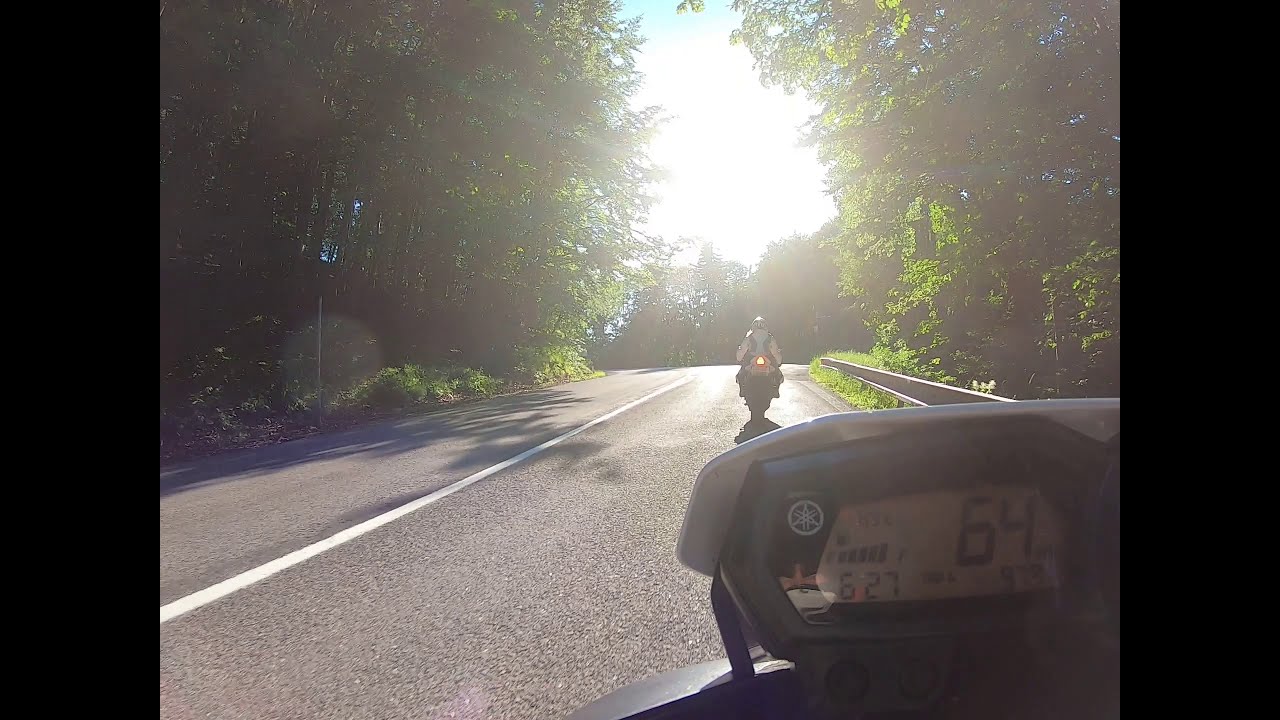This image captures a vibrant and sunny summer day on a two-lane asphalt road, flanked by tall, verdant trees forming a canopy overhead. The road is marked by a solid white line down the center and features a silver guardrail on the right-hand side. In the distance, a motorcyclist is seen riding away, their brake light or a similar rear light illuminated. They are wearing a light-colored jacket with dark trim. The photograph appears to have been taken from the perspective of another motorcycle or a vehicle, evident from a dashboard or display panel in the foreground showing the number '64,' possibly indicating the speed in miles per hour. Sunlight filters through the branches, casting a bright, almost ethereal glow over the serene, tree-lined roadway.